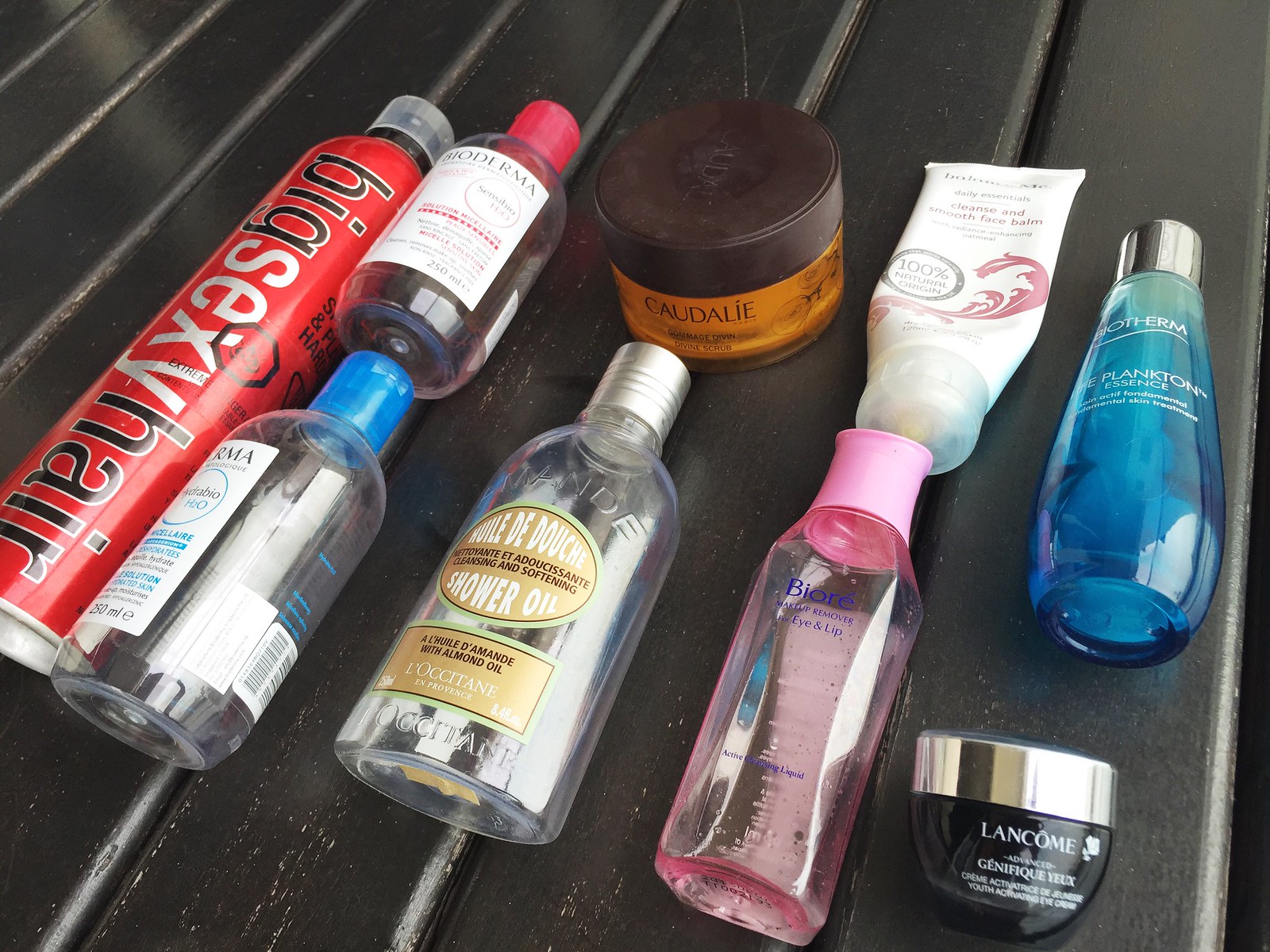A meticulously arranged display of various liquids and pastes, each housed in uniquely labeled containers, is set out on a grooved metal tray. On the left, a prominent large red bottle labeled "Big Sexy Hair" stands upright, featuring a plastic top. Adjacent to it, slightly overlapping, are two bottles bearing the "Moderna" label. One is a clear bottle with a white label and red top, potentially a shampoo, while the other is a blue bottle with a blue top, also likely a shampoo despite its label being partially obscured.

In the center of the arrangement, a large bottle divides the display into two sections, with a distinct grouping above and below it. A brown container with a dark brown top, branded "Caudalie," is positioned next to a silver-topped bottle labeled "Shower Oil." Alongside this, a clear bottle maintains the symmetry of the layout.

The next section includes a seemingly used, almost empty tube labeled "Face Balm," signifying its frequent use. Nearby, a clear bottle with a pink top appears to contain an eye care product, although the full label is partially obscured. 

Concluding this array, a pair of distinctive bottles draws attention. One, labeled "Othram Plankton Essence," is a clear bottle filled with blue liquid and capped with a silver top. The other, a small container from "Lancôme Génifique," features a sleek black base and a matching silver screw top. 

This organized collection showcases a range of personal care products, each with its unique purpose and design, meticulously placed on the tray.